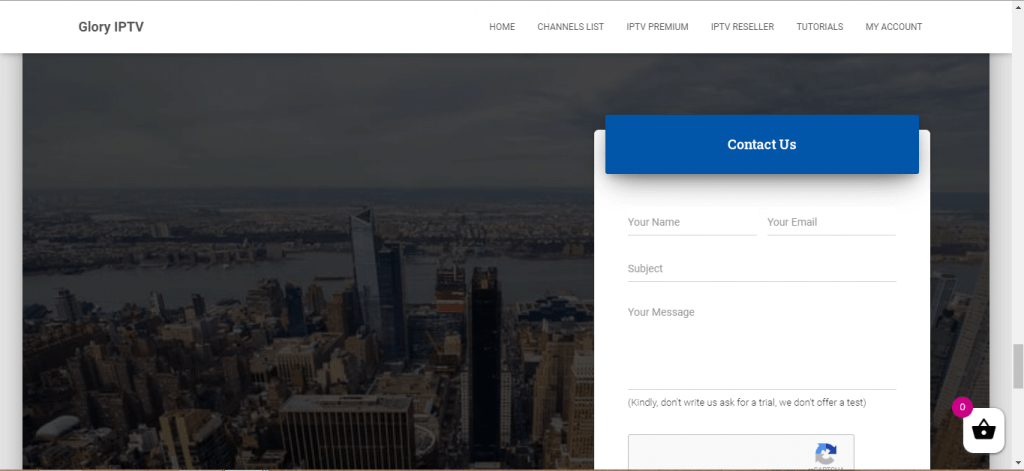The webpage for Glory IPTV is meticulously detailed on this image. On the top left, the title "Glory IPTV" is prominently displayed in black text. Correspondingly, on the top right, there are navigational tabs labeled in black. These tabs include "Home," "Channel List," "IPTV Premium," "IPTV Reseller," "Tutorial," and "My Account," providing organized access to different sections of the site.

To the right side of the page, there is a sign-up section featuring a blue "Contact Us" button with white text. This button, when clicked, allows users to reach out by filling in their name, email, email subject, and message. Beneath this form, there's a warning: "Kindly, don't write us, ask for a trial, we don't offer a test." Below this message, a reCAPTCHA checkbox is present to verify the user's human status.

Additionally, in the bottom right corner, there's a shopping cart icon highlighted in pink with a white "0" inside, indicating no items in the cart.

The background of the main page showcases an urban landscape with a combination of tall and short buildings, representing a large city. This cityscape is divided by a lake, creating a picturesque view with one city on the lower part of the image and another on the upper part.